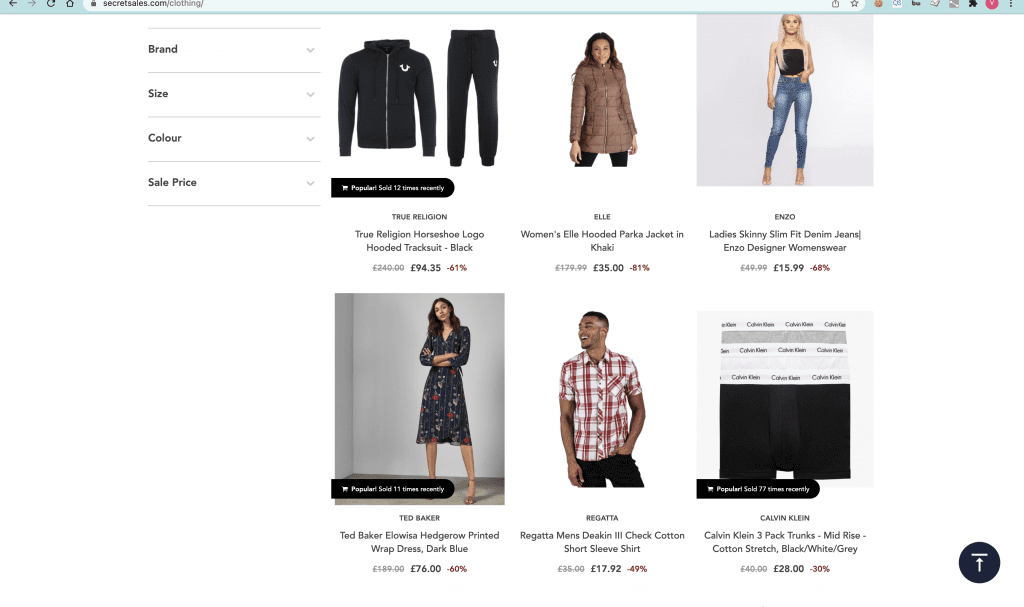This is a detailed screenshot from the clothing section of an online store, specifically the URL secretsales.com/clothing. On the left-hand side of the screen, there are sorting options available to the user, including filters for brand, size, color, and sale price, all of which are accessible via drop-down menus. 

On the right-hand side, the page showcases six different clothing items arranged in a grid format:
1. **Top Left:** A navy blue jogger set, consisting of long-sleeve top and long pants, featuring a white logo on the chest.
2. **Top Center:** A brown women's coat that extends just past the hips, offering a midway length.
3. **Top Right:** A blonde woman modeling a pair of pants and a top.
4. **Bottom Left:** A dark-color sundress adorned with floral patterns.
5. **Bottom Center:** A men's button-up flannel shirt.
6. **Bottom Right:** A black square placeholder, possibly a partially loaded image or a description, which mentions Calvin Klein, likely indicating a three-pack of trunks.